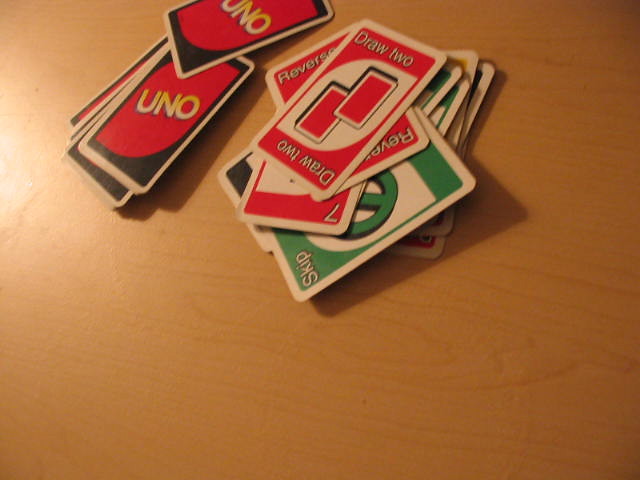In the image, there's a stack of UNO playing cards arranged in two primary piles on a light teal, smooth hardwood surface. The deck contains about 20 disheveled face-down cards, while the larger portion of the deck is face-up, indicating cards that have been played. The face-up cards showcase a variety of actions and colors, such as a red "Draw Two" card, a red "Reverse," a red number seven, and a green "Skip" positioned slightly beneath them. On the left side, there are about five or six face-down cards peeking out, adding to the disarray. On the right side, various face-up cards jut out, showing a mix of yellow, green, and red colors. The pristine playing surface highlights the intense and engaging gameplay that has unfolded, featuring skip, reverse, and draw two cards in quick succession, suggesting a competitive and strategic session of UNO.